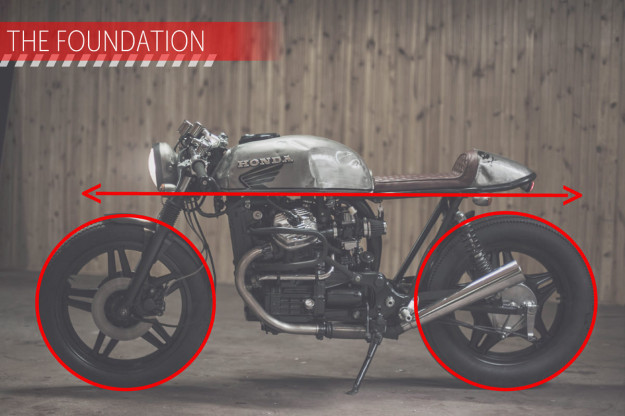The image features a Honda motorcycle set against a vertically-striped, grayish-brown wooden wall, possibly paneling or a fence. The wood has numerous darker knots that add texture to the vertical stripes running from the top to the bottom of the picture. The motorcycle is upright on its kickstand, with the front of the bike facing the left and the rear to the right. The word "Honda" is prominently displayed on the gas tank. 

Across the middle of the motorcycle, just below the gas tank and seat, runs a horizontal red line with arrow points at both ends, extending most of the width of the picture. The bike's black tires are encircled by red rings. The entirety of the image is subdued in color, with predominant tones being gray, black, white, and brown, highlighted by the striking red circles and horizontal line. 

In the upper left corner, within a red rectangle, the words "THE FOUNDATION" are written in white capital letters. The motorcycle's headlamp is illuminated on the right side, adding a touch of brightness to the otherwise grayscale aesthetic.